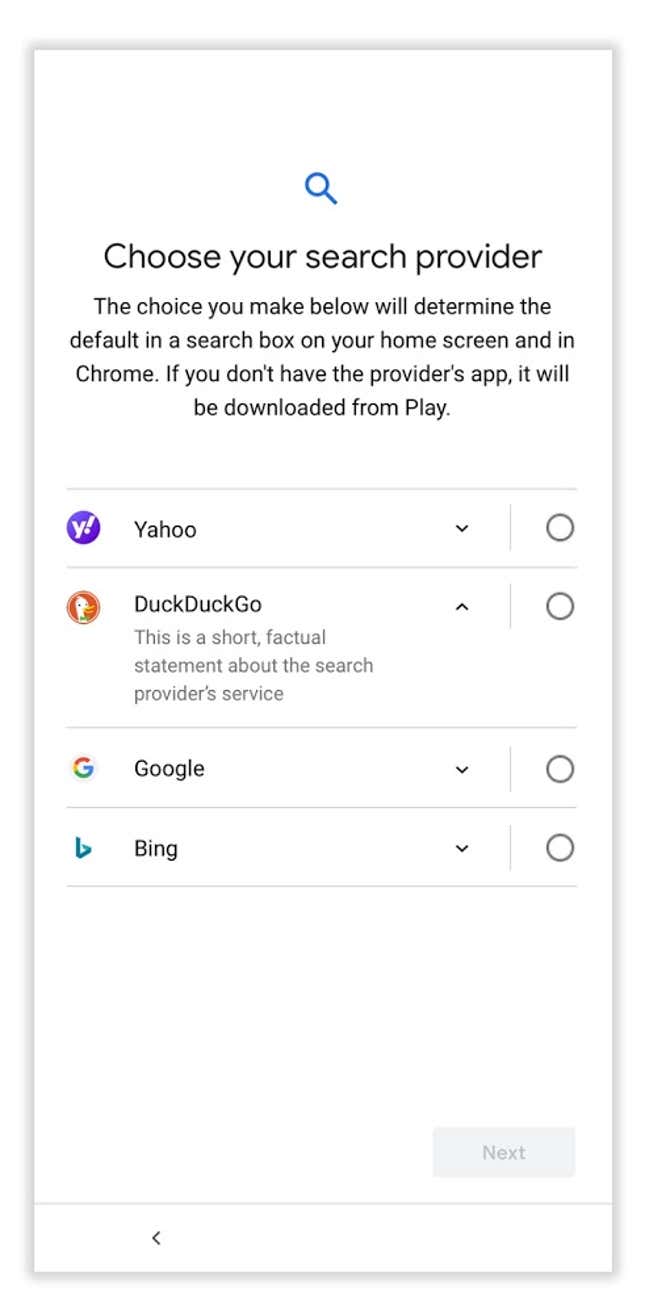The screenshot captures a phone screen displaying a user interface prompting the user to select their default search provider. The interface features a clean, predominantly white background with a blue magnifying glass icon centered near the top. Directly below the icon, in large, non-bold black text, it says, "Choose your search provider." Following this, a smaller text in the same font explains, "The choice you make below will determine the default in the search box on your home screen and in Chrome. If you don't have the provider's app, it will be downloaded from Play."

Beneath this explanatory note, a list of search engine options is presented. Each option is accompanied by its respective logo to the left and a selection bubble to the right. The options include:

1. **Yahoo** – with the Yahoo logo.
2. **DuckDuckGo** – coupled with a factual statement describing the service.
3. **Google** – accompanied by the Google logo.
4. **Bing** – with the Bing logo.

As of now, no search engine has been selected, although DuckDuckGo's informational text stands out, perhaps drawing curiosity from the user. To finalize their choice, the user can press the "Next" button located in the lower right-hand corner of the screen.